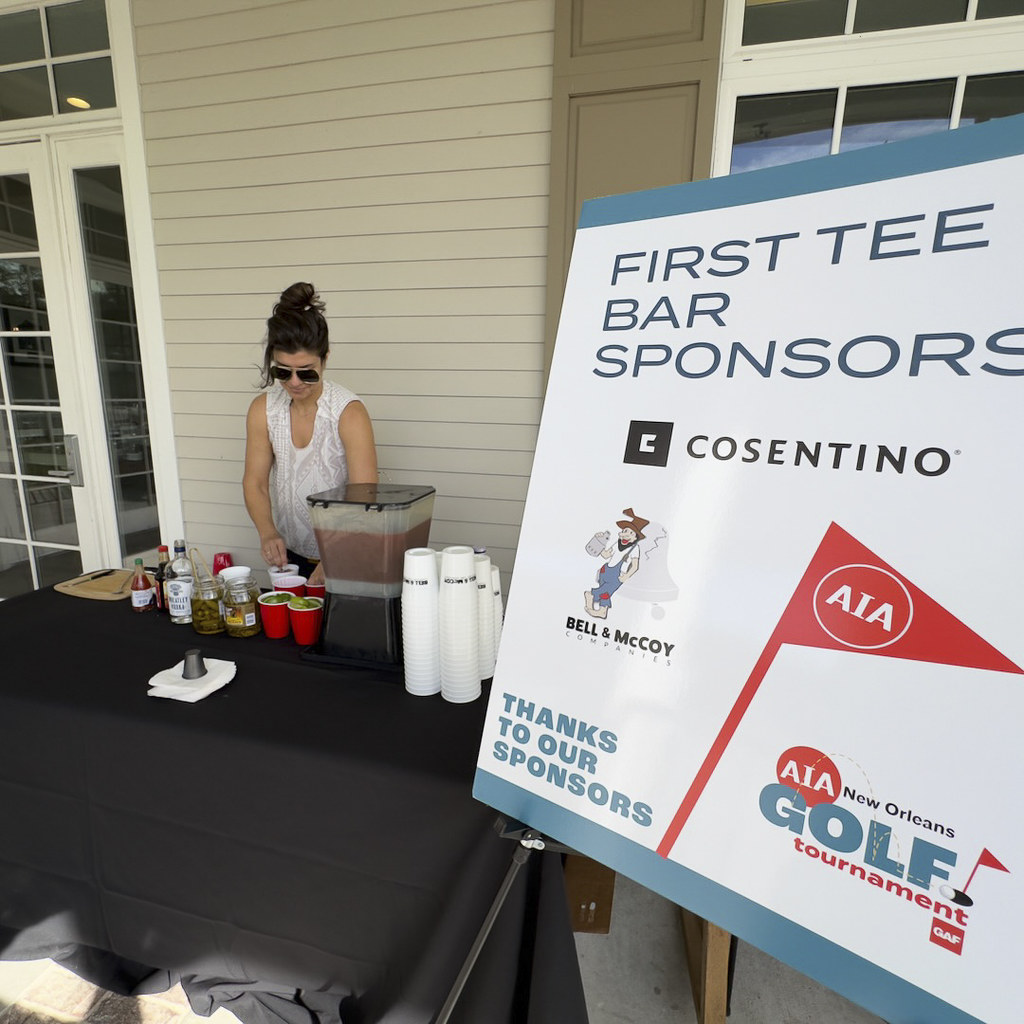This image captures an outdoor scene at a golf tournament, where a young woman stands behind a small food and beverage stand set against a building with an open doorway on the left. The woman, dressed in a sleeveless white shirt and sunglasses, is likely serving refreshments. On her stand, there's a large juicer or mixer surrounded by a variety of items: neatly stacked white plastic cups to its right, red cups filled with what appears to be pickles or limes to its left, and several open jars of pickles. Additional condiments and a cutting board are also present further to the left. A shaker cup rests on a towel in front of all these items, suggesting she might be preparing drinks, possibly including alcohol as hinted by a visible bottle. Dominating the right side of the scene, a detailed sign reads "First Tea Bar Sponsors," listing sponsors like Cosentino, Bell & McCoy, and acknowledging AIA New Orleans Golf Tournament, indicating that this stand is part of the event.